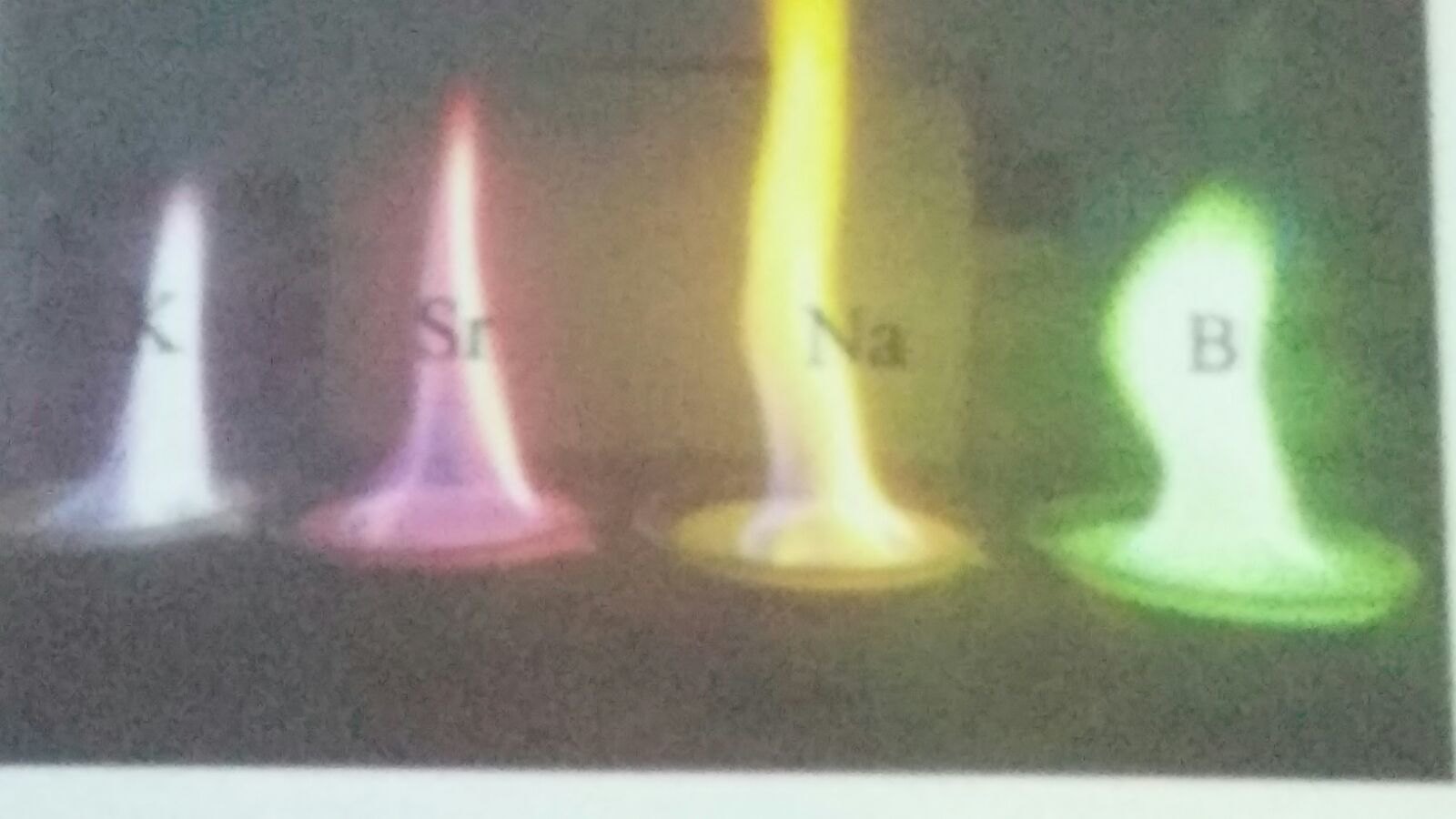The image depicts a scientific experiment featuring four small frames, each set on a circular base and emitting distinct colored flames. The overall image is grainy and blurred, set against a brown, blurry background. On the far left, there's a white frame with a black letter 'K,' mounted on a circular base, which emits a bluish-white flame. Next to it, a pink frame on a matching circular base displays the letter 'S' and has a pinkish-purple flame. The third frame is the tallest, yellow with the symbol 'NA' and a yellow flame. On the far right, a green frame with a capital letter 'B' on its green circular base produces a green flame. The entire setup hints at a scientific context, potentially a chemistry demonstration.